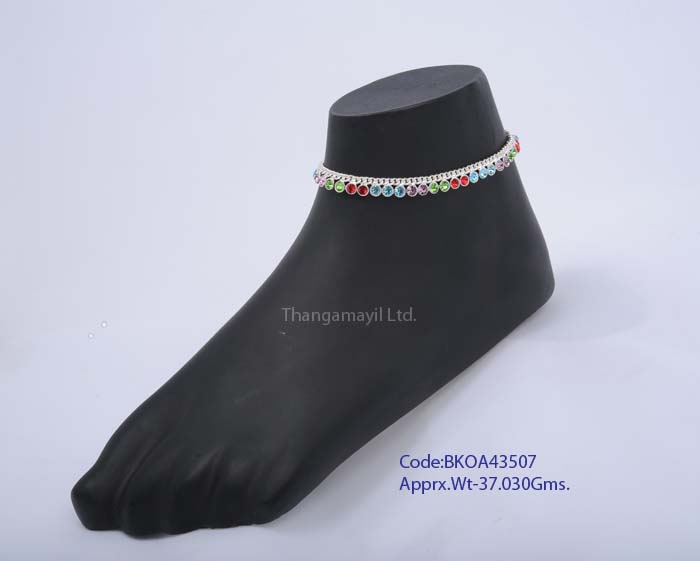A detailed photograph depicts a black mannequin's foot positioned diagonally on a white background, with the toes oriented towards the bottom left corner and the heel pointing to the top right. The mannequin foot is severed at the ankle, showcasing a smooth, flat top. Adorning the ankle is a delicate silver anklet, featuring a thin chain and a multitude of colorful crystals, including green, red, blue, purple, and orange, each encased in silver and hanging daintily. The anklet's display is the focal point of the image. Embellished details include “Thangamayil Ltd” in white lettering in the center of the image and an annotation in dark blue in the bottom right corner, stating "CODE BKOA43507," with an approximate weight of 37.030 grams.